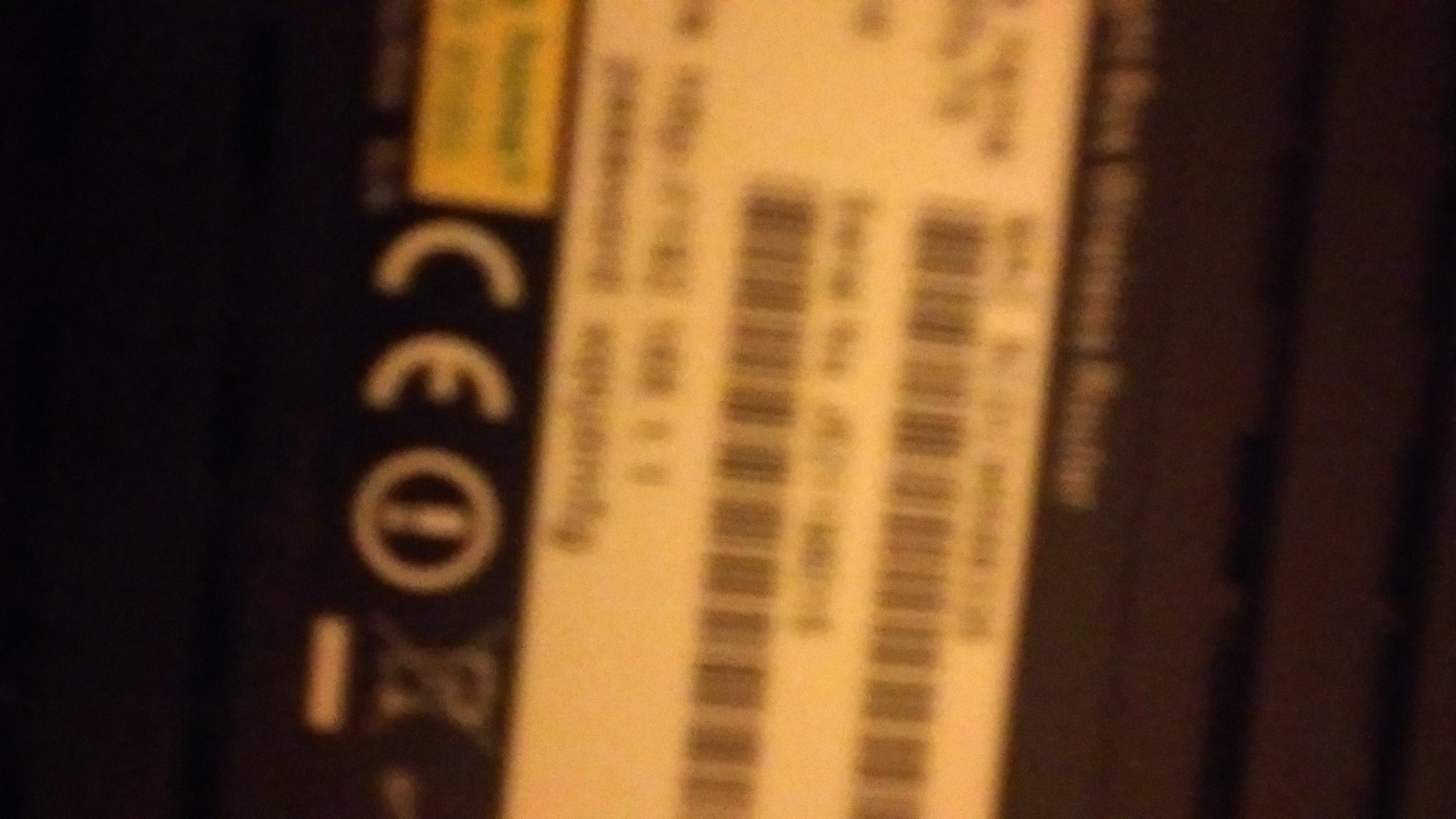This close-up image, likely taken with a phone camera, depicts the underside of a wireless router. The image is primarily focused on a white label affixed to the router, which contains two barcodes. One barcode is likely the serial number of the router, while the other may serve as inventory identification for the Internet Service Provider (ISP) that issued the device. Additionally, a smaller yellow label can be seen on the white label. The white label also features several regulatory marks, including the CE mark, which signifies compliance with European safety, health, and environmental requirements. The photo is notably blurry, rendering most of the text and details on the labels unreadable.